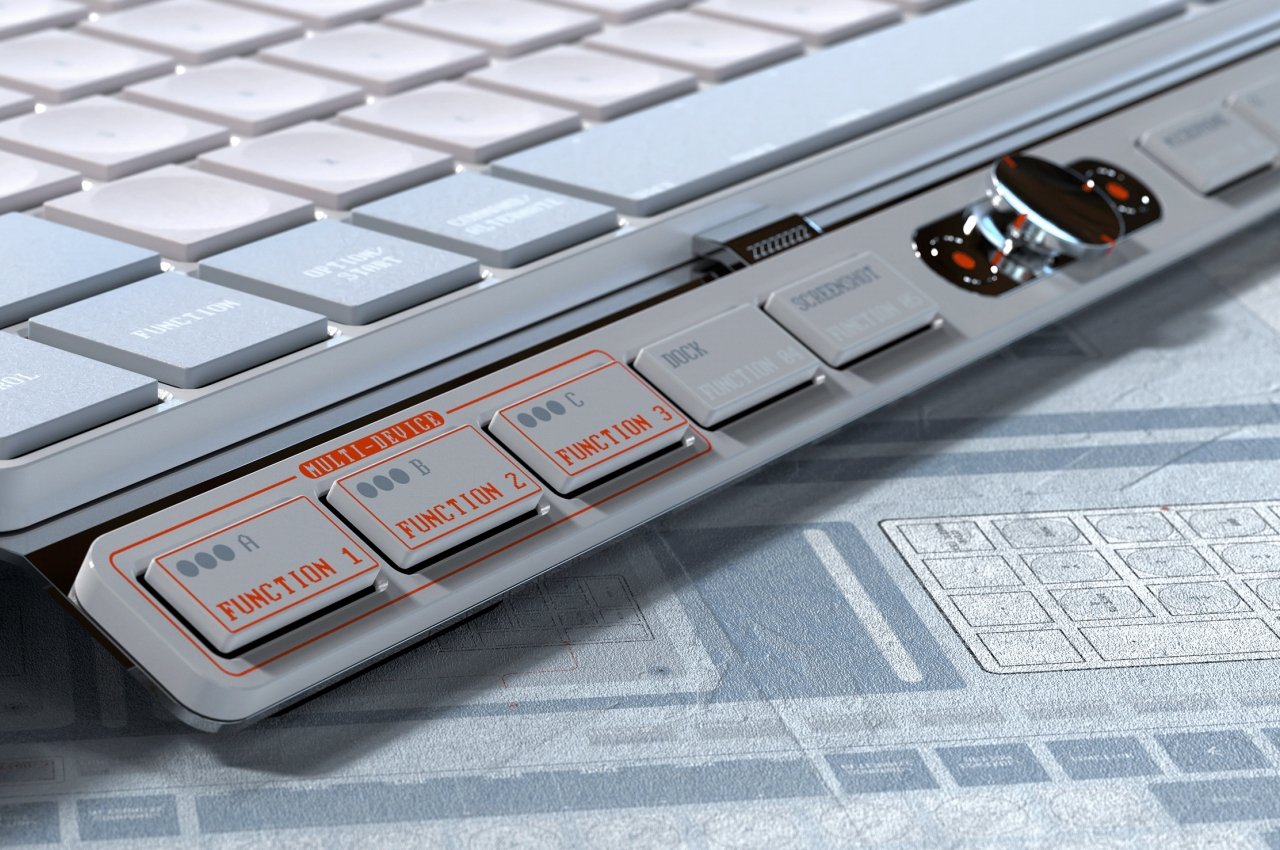This close-up photograph depicts a non-standard, gray and white keyboard, positioned at an approximately 45-degree angle atop a surface that appears to have an instructional sheet beneath it, showcasing the same keyboard. The keyboard's main keys, predominantly white with some light blue around the spacebar area, are complemented by an add-on section at the bottom with distinct features. This bottom extension includes three buttons labeled "Function 1," "Function 2," and "Function 3," each surrounded by a thin orange outline and three gray circles marked "A," "B," and "C" respectively, indicating possible LED indicators. Additionally, there are keys labeled "Dock" and "Screenshot," and the overall outline of the extension is accented by an orange line. The term "multi-device" is inscribed at the top of this section. The photograph also highlights a metallic component slightly tilted to the right, suggesting part of the electronic mechanism. This unique keyboard layout is detailed in the underlying printed diagram, which further illustrates its functional mapping.